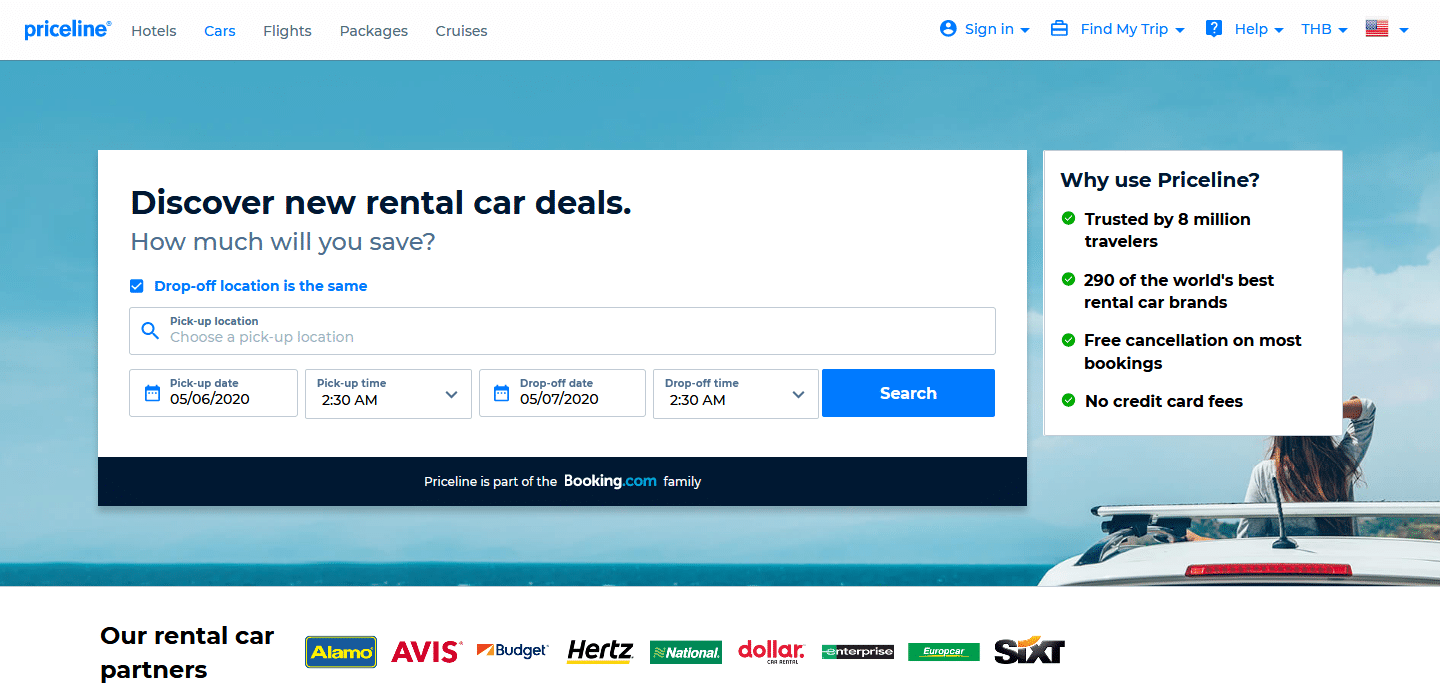The screenshot from the Priceline website features a well-organized interface designed to facilitate rental car bookings. In the top left corner, the Priceline logo is displayed in lowercase blue letters. The main menu bar includes options: Hotels, Cars (currently selected), Flights, Packages, Cruises, Sign In, Find My Trip, Help, THB, and an icon representing the American flag. 

In the background, a serene photograph captures the horizon under a partly cloudy blue sky. A woman sits inside a white convertible, facing away from the camera, positioned in the bottom right corner of the image, likely enjoying the view.

Dominating the center, a prominent white rectangle encourages users to "Discover New Rental Car Deals" and asks, "How much will you save?" The pre-selected option indicates that the "Drop off location is the same." It also prompts users to choose a pick-up location, with default pick-up and drop-off dates set to May 6 and May 7, 2020, respectively, both at 2:30 AM. A "Search" button is available for users to initiate their booking inquiry.

Just below the main section, a black banner declares, "Priceline is part of the Booking.com family." Adjacent to this, a white square offers compelling reasons to use Priceline: it is trusted by 8 million travelers, partners with 290 of the world's top rental car brands, provides free cancellation on most bookings, and charges no credit card fees.

At the very bottom of the webpage, the logos of Priceline’s rental car partners are displayed, including recognizable names such as Alamo, Avis, Budget, Hertz, National, Dollar, Enterprise, Europcar, and SIXT.